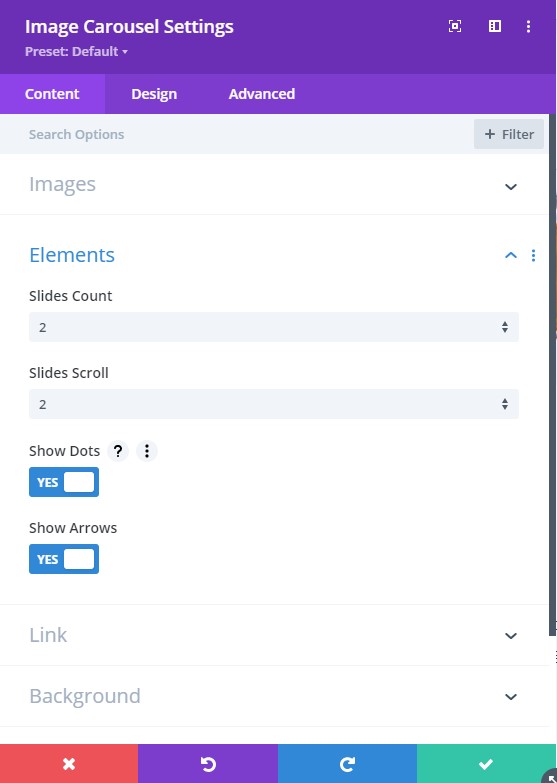In this image, we see an interface that appears to belong to a settings menu for a computer program or application, specifically tailored for configuring an image carousel. At the top, there is a purple header with the title "Image Carousel Settings" in white font. Adjacent to this header are a couple of square icons, though their functions are unclear.

Immediately below the header, there's an option labeled "Preset: Default." Further down, there are three main tabs: Content, Design, and Advanced, each likely providing different categories of settings. Within this section, we also find sub-tabs labeled "Search Options" and "Images," both highlighted in red and gray. 

Under the "Images" tab, we have additional sections described as "Elements." Below this, there are labels for "Slides Count" and "Slides Scroll," each displaying the number 2. The interface then offers clickable toggles for "Show Dots" and "Show Arrows," both of which are switched to "Yes."

At the bottom of the interface, there are further setting options for "Link" and "Background," suggesting customization capabilities for these elements within the image carousel. This comprehensive setup provides users with various tools to configure the visual and functional aspects of an image carousel effectively.